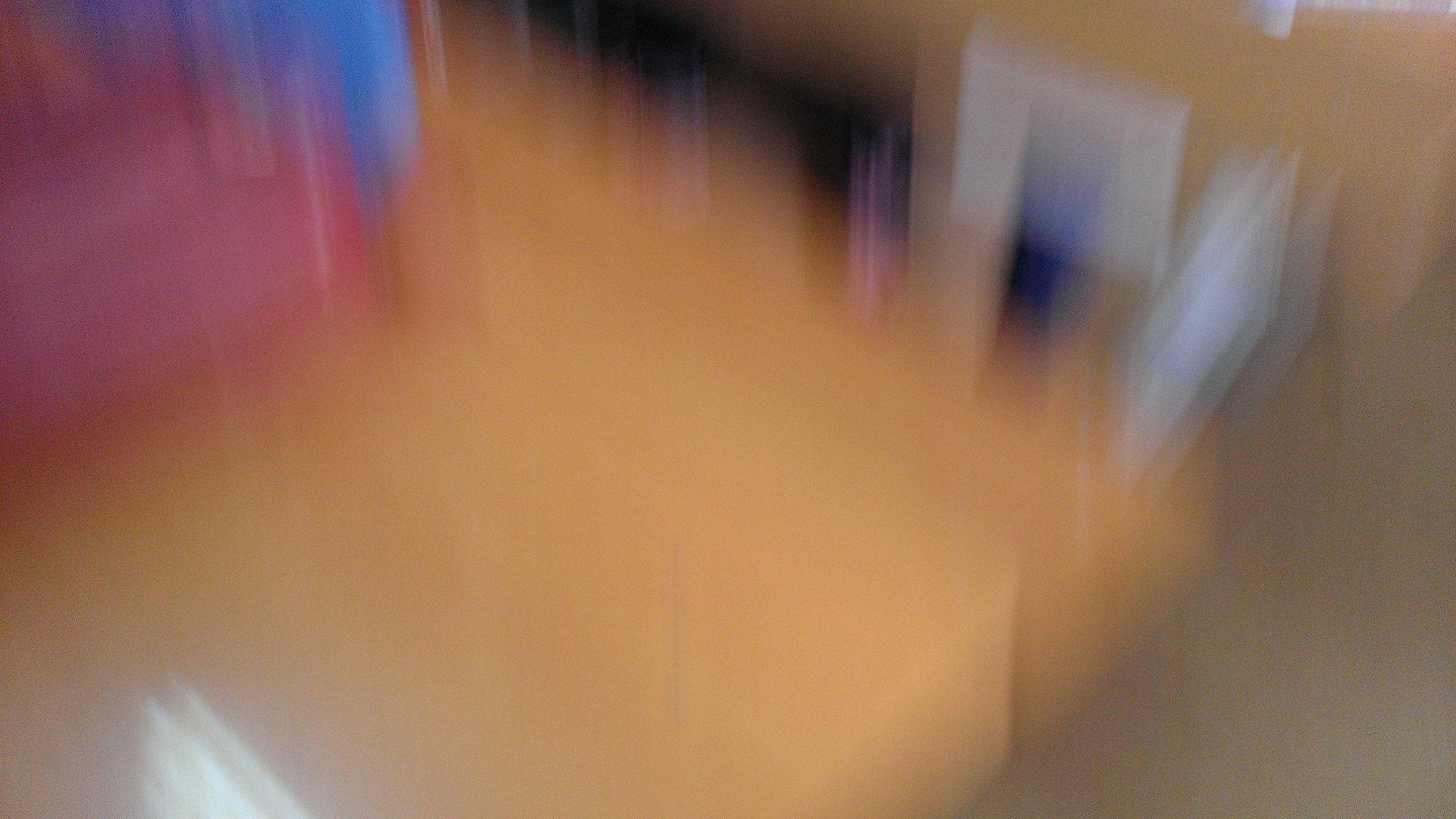This blurry image features an abstract composition of various shades and colors. Starting at the top left-hand corner, there is a blend of maroonish pink and blue hues. Below this, an abundance of orange tones forms what appears to be a cubicle-like shape. Adjacent to the maroon red, a bright white reflection is noticeable toward the bottom left-hand corner. 

In the center at the top, a combination of dark purple, black, and light pink colors dominates the scene. To the right of this, multiple square-shaped flashes of light, primarily white with a purple center in one of them, add a striking effect. The bottom right-hand corner transitions into a darker peach shade, eventually melding into a gray tone. Overall, the image presents a complex and indistinct mixture of colors and shapes.